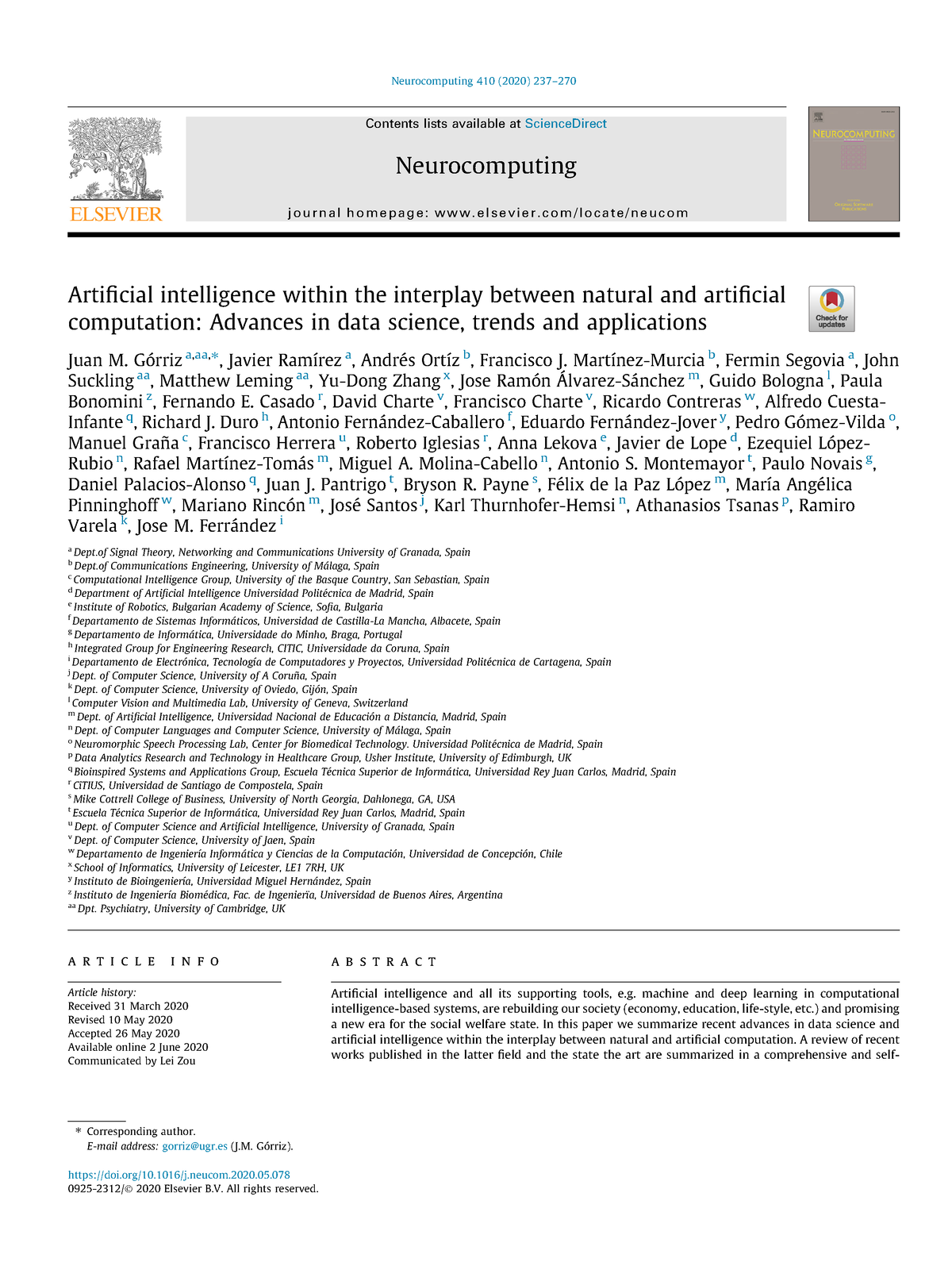A low-resolution, cropped screenshot of a website displays content primarily in black text on a white background, making it challenging to interpret many details. At the top of the image, a gray banner reads "Neurocomputing," with additional text below it that is largely illegible, except for a possible URL and some words like "contents available" and "ScienceDirect." Above the gray banner, blue text resembling a hyperlink includes numbers and a date. To the left of this banner is an icon or logo of a tree followed by the word "Elsevier" in orange text. To the right, a dark gray box contains yellowish hyperlinks, which are also unreadable due to the resolution.

Following the banner is a title, "Artificial Intelligence within the Interplay between Natural and Artificial Computation: Advances in Data Science, Trends, and Application," accompanied by a long list of names, many of which appear to be Hispanic. Below the title, there seems to be a block of black text, likely citations, but it is too pixelated to decipher.

Underneath this block, the section labeled "Article Info" features a small table of details that are similarly unreadable. To the right of this table, the abstract section begins, where only a few words such as "artificial intelligence" and "AI" can be distinguished. At the bottom left, additional indiscernible text is present alongside two blue hyperlinks, one of which is notably longer than the other.